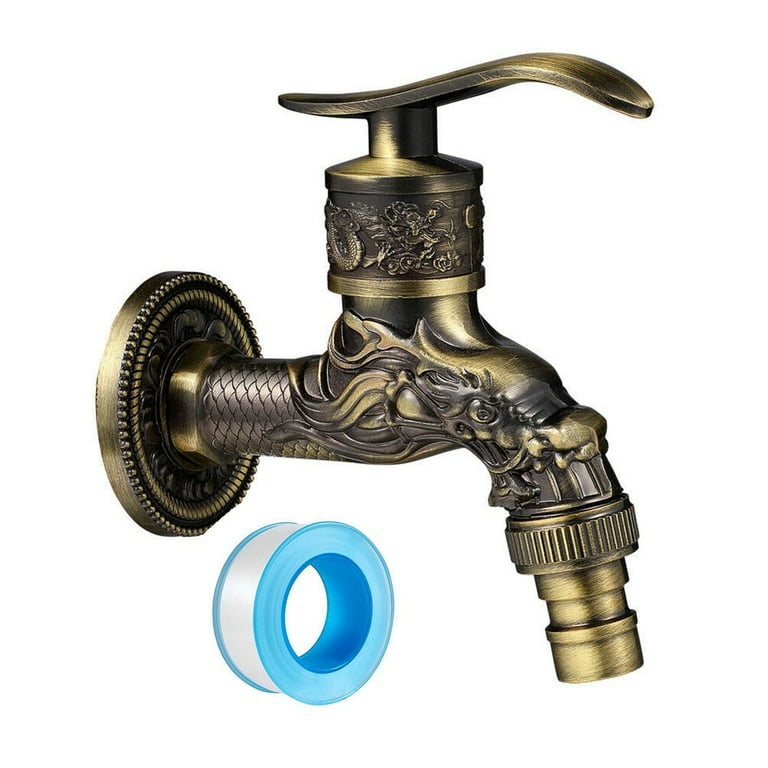This is a detailed product image of an ornate water spigot designed to resemble a dragon, set against a white background. The spigot, which appears to be made of brass or an antique gold finish, showcases an exquisite level of craftsmanship. The main body of the spigot is sculpted to feature dragon scales, with the water flowing out from the mouth of a highly detailed dragon head. The spout connects to the water line via a circular medallion-shaped base, intricately etched with scallops and scroll-like designs to mimic dragon scales. Above the dragon head, there's a column-like section capped with a large, wavy handle for turning the water on and off, adorned with a smaller ornamental dragon figure just below it. Complementing the spigot's luxurious aesthetics, there is a blue plastic spool containing white Teflon tape, presumably for installation purposes, visible beneath the spout in the photograph.